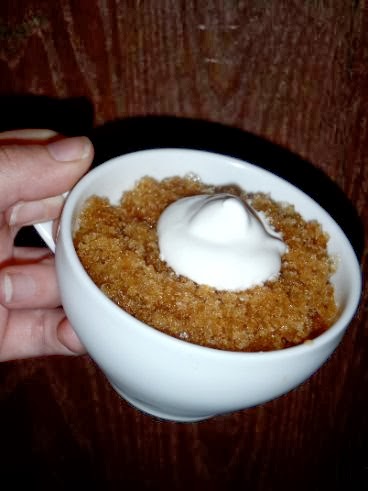A photograph features a left hand with light, fair skin, and closely trimmed, bare fingernails, holding a white ceramic mug by its handle. Inside the mug is an orange, crumbly dessert, topped with a dollop of whipped cream forming a peak. The mug casts a dark shadow onto the background. This background consists of a dark brown wooden surface with visible wood grain, which could be either a wall or a table.